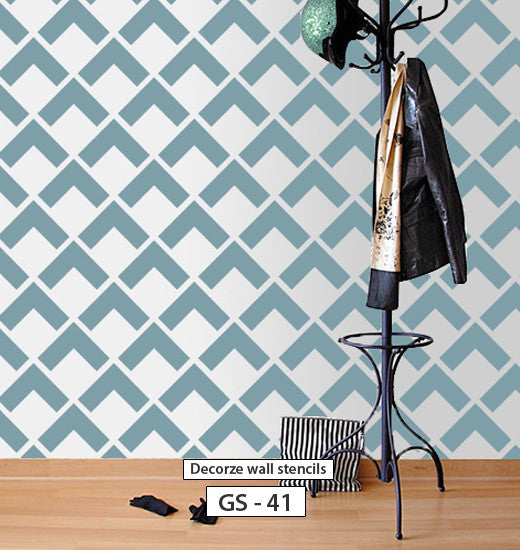This detailed image captures a black metal coat rack standing on a light tan wooden floor. The coat rack has a tripod base connected to a circular holder, possibly for an umbrella. Moving upward, it features a series of smaller hooks followed by larger ones. A black leather coat with what looks like gold lining and an ivory-colored scarf is draped over the smaller hooks. Topping the rack is a helmet, potentially used for skateboarding, colored in a greenish hue with a golden sparkle. Surrounding this setup, a striped black and white handbag rests on the floor next to a pair of black gloves. The backdrop is a white wall adorned with a light blue geometric design, resembling three-dimensional boxes in a stenciled pattern. At the bottom of the image, two white boxes contain the text "Decorus Wall Stencils" with the number "GS-41," likely indicating the stencil pattern used for the wall design.